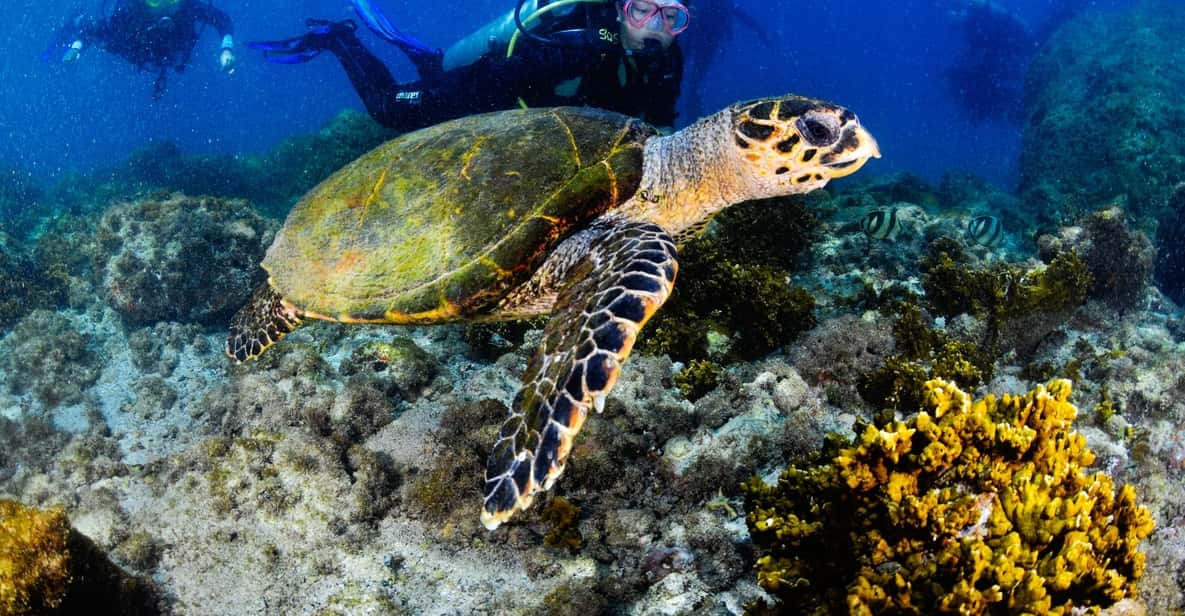In this captivating underwater scene, a prominent sea turtle swims gracefully in the foreground. This mature sea turtle, recognizable by its large size and the green moss growth on its black, leathery shell, features scaly fins and an outstretched neck, revealing a slightly beaked mouth and a large, dark eye. The background transitions into a darker blue hue, highlighting the turtle under the lit water. Below this majestic creature, the ocean floor is adorned with a variety of colorful corals, underwater plants, and scattered rocks.

The scene is further enriched by the presence of several scuba divers exploring the marine environment. Directly behind the sea turtle is a female diver, easily identifiable with hot pink goggles, a light-colored air tank, and a dark scuba suit. Her hair floats freely in the water. To the left, slightly detached from the group but moving towards the turtle, is another diver with yellow goggles, swimming with curiosity towards the view. The interplay of marine life and human exploration captures a vivid snapshot of underwater adventure.